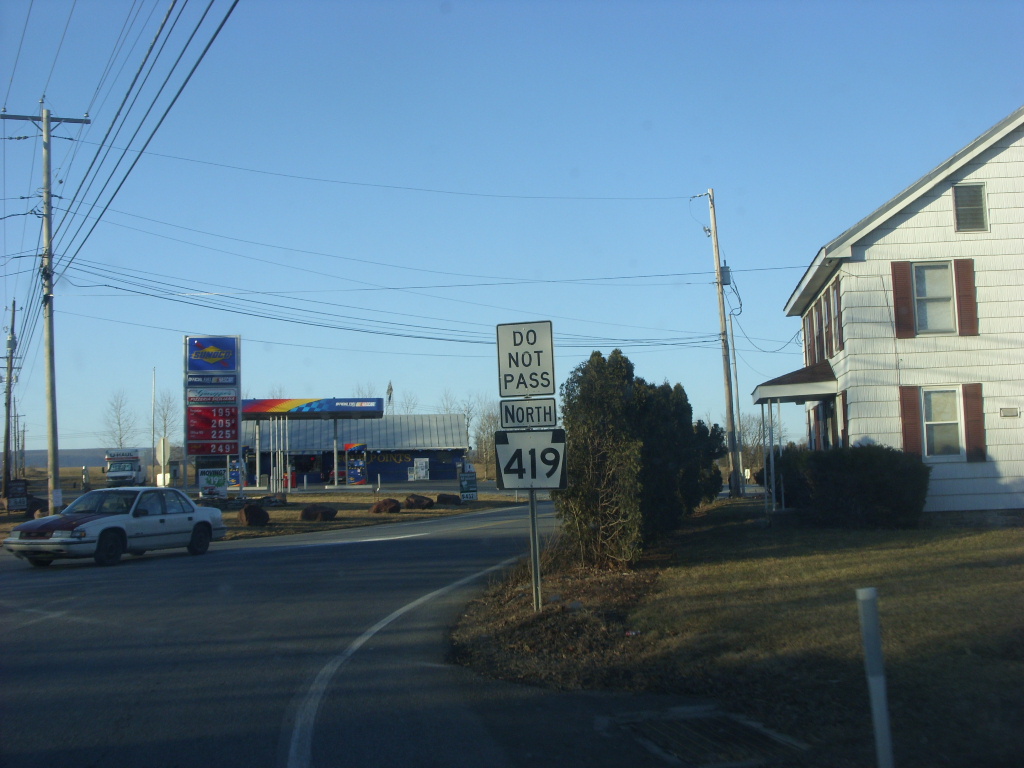The photograph captures a rural road that curves to the right, with a white safety line marking its edge. On the right side of the road stands a white house with brown shutters on both floors and a covered porch flanked by hedges. The road comes up to the house's lawn, lacking any sidewalk. The driveway adjacent to the house reveals more hedges and trees lining the roadside.

Prominent in the middle of the image are three white street signs on a single pole, displaying "Do Not Pass," "North," and "419," indicating the highway number. Additionally, power lines and telephone poles are visible, running along the road's curve.

On the left side of the image, a blue Sunoco gas station with a distinctive red, yellow, and blue design on its fuel pumps stands out. The gas prices on the large vertical sign read $1.95, $2.05, $2.29, and $2.49. Positioned in front of the gas station is a U-Haul truck.

The foreground of the image highlights a small white car with a contrasting brown hood, likely a model from the 1980s or 1990s, heading south down the road. Trees without leaves diffuse into the background, adding to the rural ambiance.